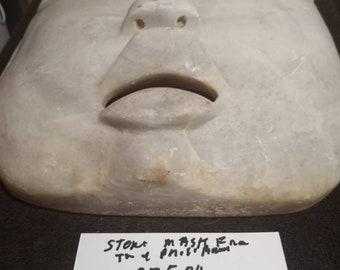The image displays an ancient artwork of a stone mask positioned centrally and slightly upwards, revealing its contours and intricate design. The mask, presumably crafted from a whitish-gray stone resembling granite with faint veining, presents a detailed yet eerie facade. Its expression is captured with a subtly open mouth, showcasing flat lips with a ledge underneath, and a nose that is broad and flat with visible nostrils. The mask extends from the chin to just above the nose, leaving the eyes out of view, which adds to its mysterious appearance. Surrounding the mask is a varied palette of grays, whites, blacks, and pale dingy yellows, set against what looks like a table. Below the mask, a sign with scribbly handwriting reads "stone mask FNA," though the rest of the text is illegible. This carefully positioned artifact exudes an aura of historical significance, reminiscent of creations made hundreds of years ago.